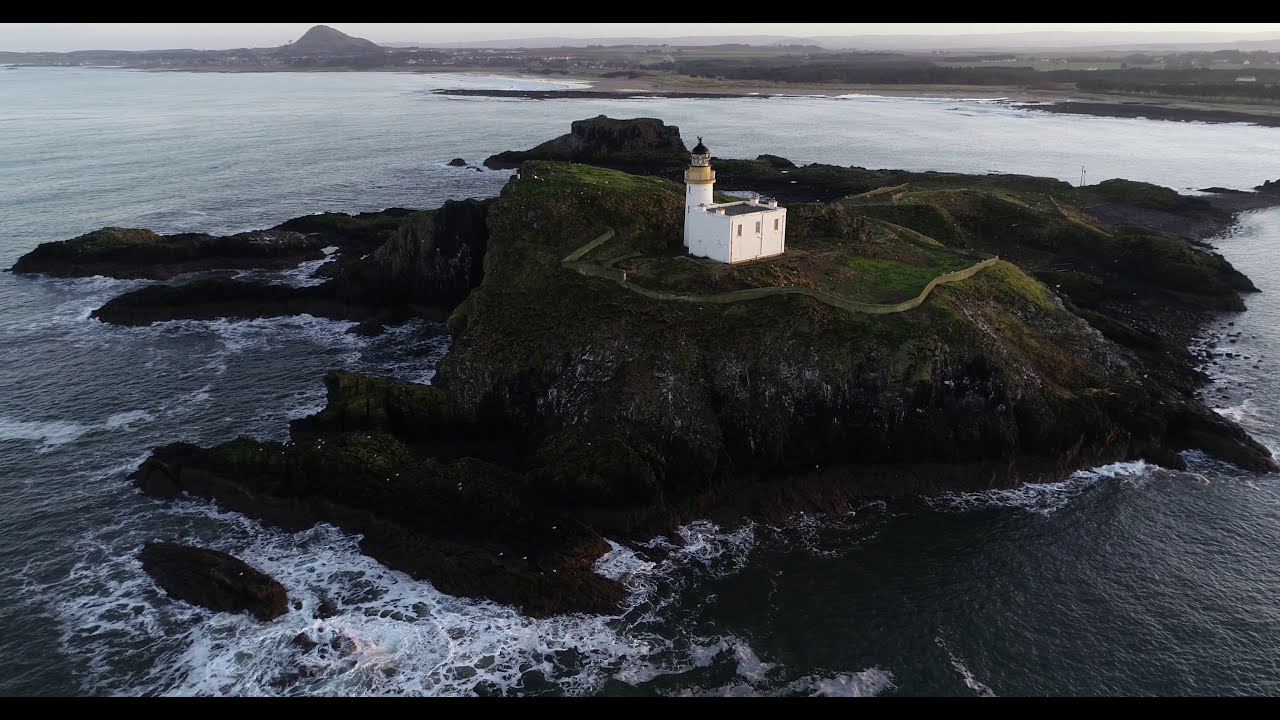This captivating image, taken during the daytime from an aerial perspective, showcases a small, rocky island rising dramatically from the ocean. The island is characterized by steep, rugged cliffs that descend into the choppy, white-capped waves, particularly visible in the lower left corner of the frame. A single notable structure, most likely a lighthouse, dominates the island’s landscape. Made of white stone, the structure consists of a large square building, probably serving as living quarters, with a lighthouse tower attached to its left. The building is enclosed by a sturdy stone wall that stands at the edge of the cliff, enhancing the island's remote and inaccessible appearance. Surrounding the lighthouse is nothing but the rugged, rocky shore, emphasizing the isolation and serene beauty of the setting. In the background, at the very top of the image, additional landmasses are visible, shrouded in a faint mist, hinting at nearby civilization. The expansive ocean encircles the island, and no signs of human or animal presence can be detected in the tranquil, almost ethereal scene.